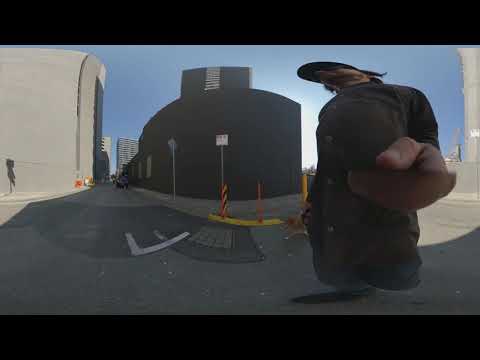A man wearing a black trench coat, resembling the WWE wrestler The Undertaker, stands in an outdoor setting, taking a selfie with a selfie stick. He appears in an abandoned parking garage, surrounded by various gray buildings on a clear blue sky day. A mirror in the scene shows his hand appearing disproportionately large as it reaches towards the camera. His head is tilted, sporting a baseball cap. To the left, a yellow-painted curb is visible along with some white road markings and a sign with yellow and black stripes halfway up. There is a light gray building in the back left corner and another dark gray building in the center. On the right, a white stone building stands. Two signposts with signs and yellow poles are along the road, and the letter "F" is marked on the ground. The sun is partially obscured by one of the buildings.